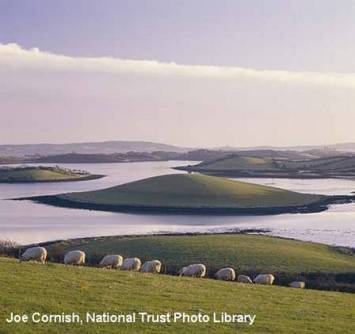The square photograph captures a tranquil rural landscape characterized by rolling green grass and a serene body of water. In the foreground, a diagonal expanse of short green grass hosts a row of approximately 10 to 12 white sheep, all appearing to graze while moving towards the left side of the image, descending a slight incline. The mid-ground features a large, still lake with a murky grayish-blue hue, providing a soft mirror of the sky above. Dominating the center of the lake is a small, rounded island, topped with lush green grass and an indiscernible object at its apex. The background reveals more of the same still waters, with additional grassy mounds or knolls scattered throughout, creating a picturesque scene. The horizon is adorned with a solitary line of white clouds, stretching across a gradient sky that transitions from bluish to purple-pink hues. Notably, the lower right corner of the image is marked with the text "Joe Cornish National Trust Photo Library," providing information about the photograph's origin.